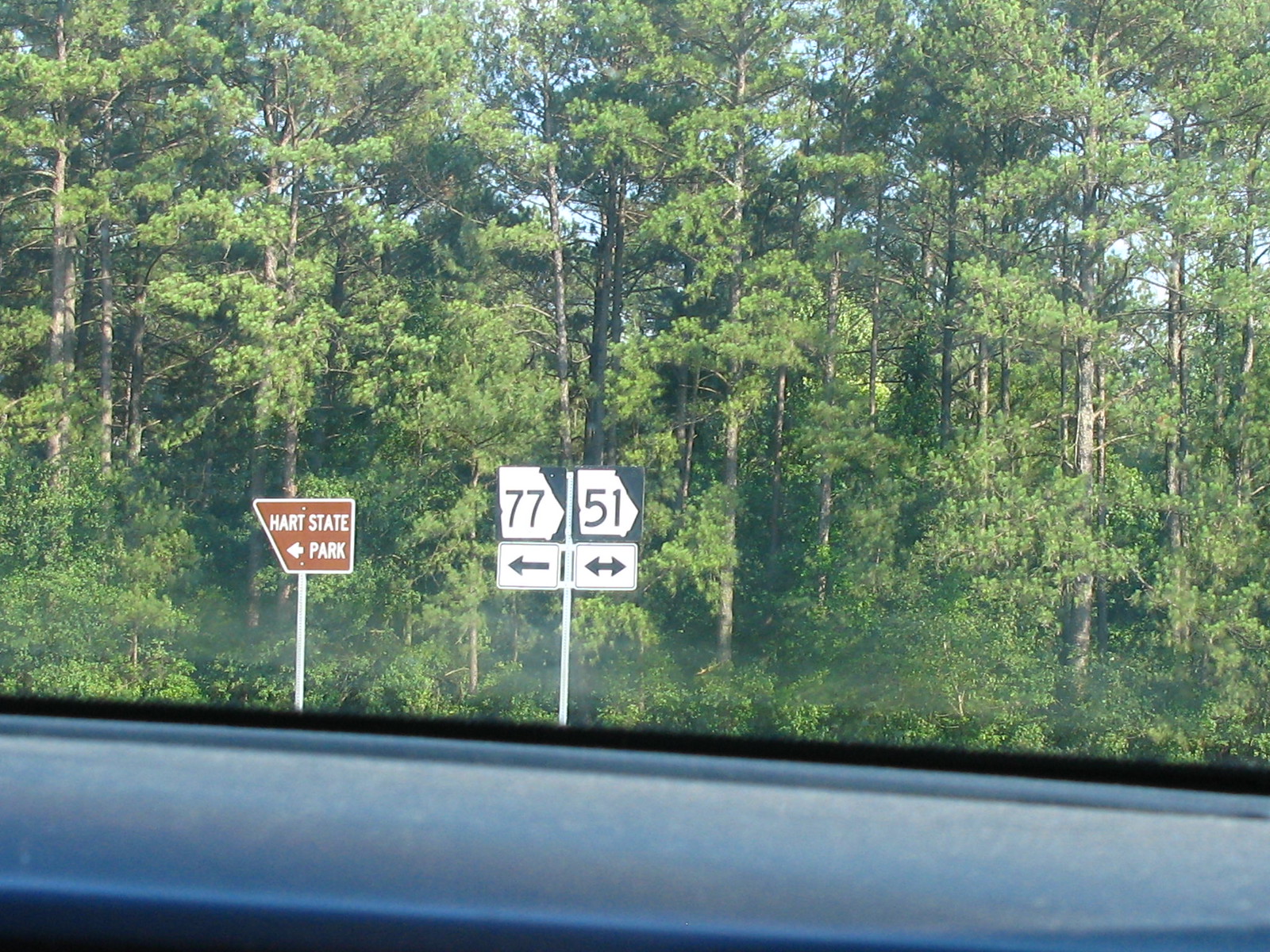In this photograph taken from the interior of a vehicle with a light blue or gray dashboard, a collection of signs and lush greenery can be seen through the windshield. At the top of the image, a brown sign clearly indicates "Hart State Park" with an arrow pointing to the left. Directly beside it, white and black interstate signs designate directions for I-77 and I-51, also featuring arrows. Behind these signs, a dense assembly of tall, green trees provides a natural backdrop, with occasional light brown tree trunks visible through the foliage, enhancing the scene's vibrant, outdoor atmosphere.